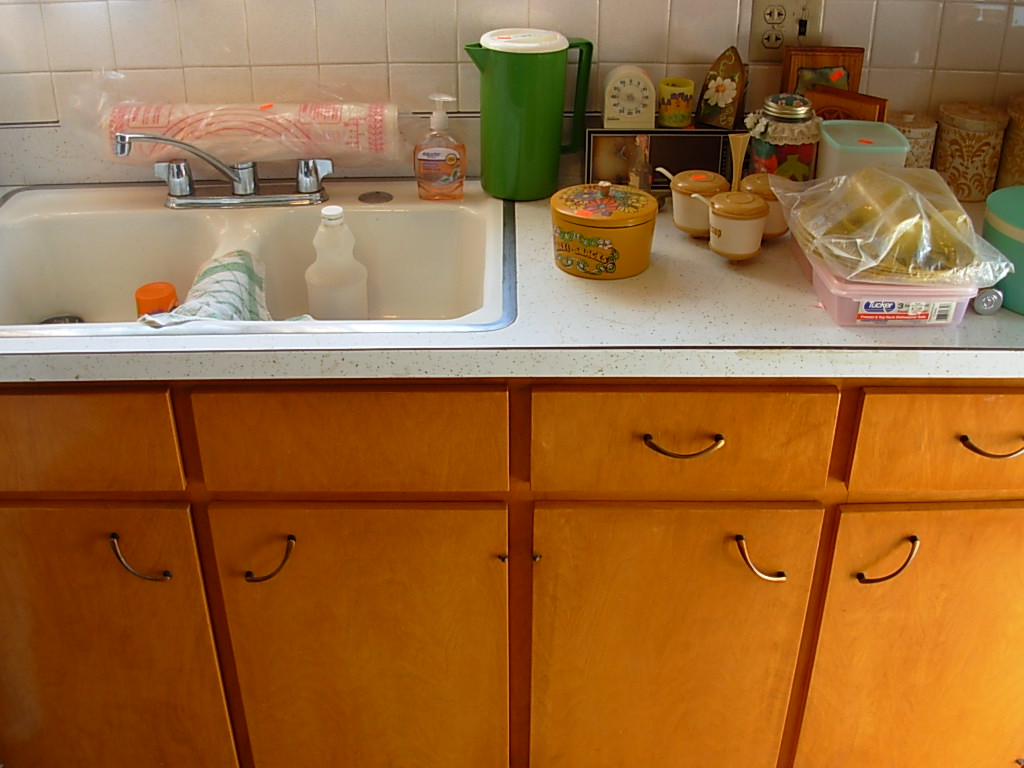A detailed portrayal of a kitchen counter and sink area reveals a harmonious blend of utility and aesthetic. Occupying the left side of the counter is a metal sink unit, its basins rendered in a dual-tone palette of white and off-white. Draped elegantly over the central divider is a white washcloth adorned with a subtle medium-green pattern. In the left basin rests an inverted orange cup.

Adjacent to this setup, an almost-empty dish soap container with a white cap sits strategically on the right side of the sink. Balanced atop the faucet is a rolled-up item, possibly a placemat, distinguished by its white base and red design.

Continuing towards the right, an orange Equate soap dispenser marks the transition to a dark green pitcher topped with a white lid. Beside it, an archetypal kitchen timer flaunts its white form, accentuated by black lettering.

In the foreground lies a mustard-yellow canister, likely for cookies or crackers, decorated with a green and white design and an orange ribbon sporting black text. Further right, a collection of small white containers with light or dark brown tops and matching writing catch the eye. Nearby, an item encased in plastic sits atop a Tupperware piece.

At the counter’s far end, an assemblage of glass or porcelain jars, featuring an orange motif and wooden lids, completes the array. The cabinetry showcases an orange wood-like hue, intensifying to a profound red in the background. The sleek, metal handles curve elegantly, while those on the lower cabinets are inclined inward, adding a touch of sophistication to the room's rustic charm.